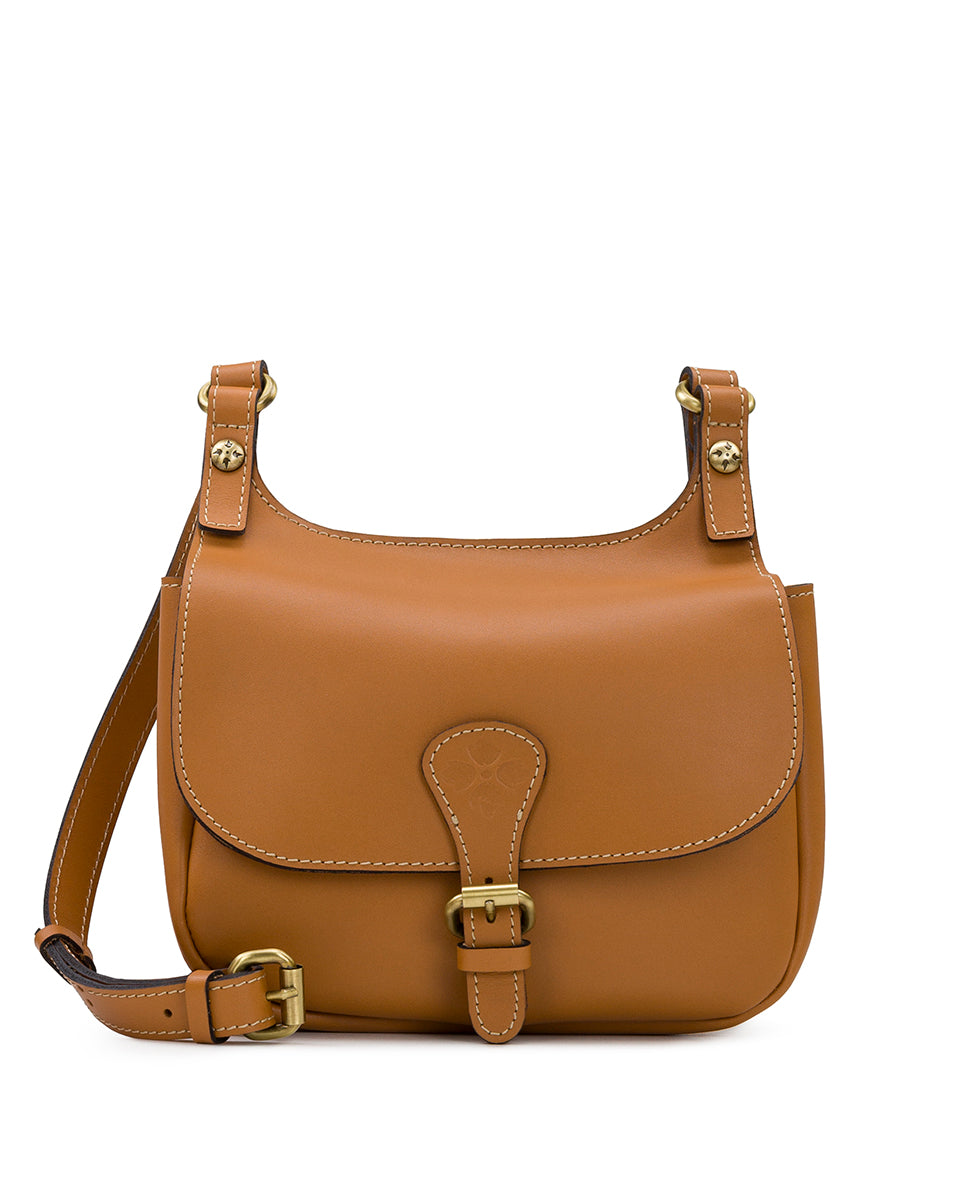This professional photograph showcases an elegant, light brown leather handbag prominently displayed against a clean white background, lending it an ad-like quality. The bag, almost square in shape with gently curved flaps, features intricate off-white stitching that highlights its craftsmanship. The main compartment, accessible through a single large flap, is secured with a distinctive brass belt buckle clasp. The strap also integrates brass buckles, adding to the bag's refined look. Two buttons and leather flaps at the top corners of the bag provide additional detailing, giving it a sophisticated yet practical aesthetic. Ideal for everyday use or a stylish exploration, this handbag combines both function and fashion seamlessly.